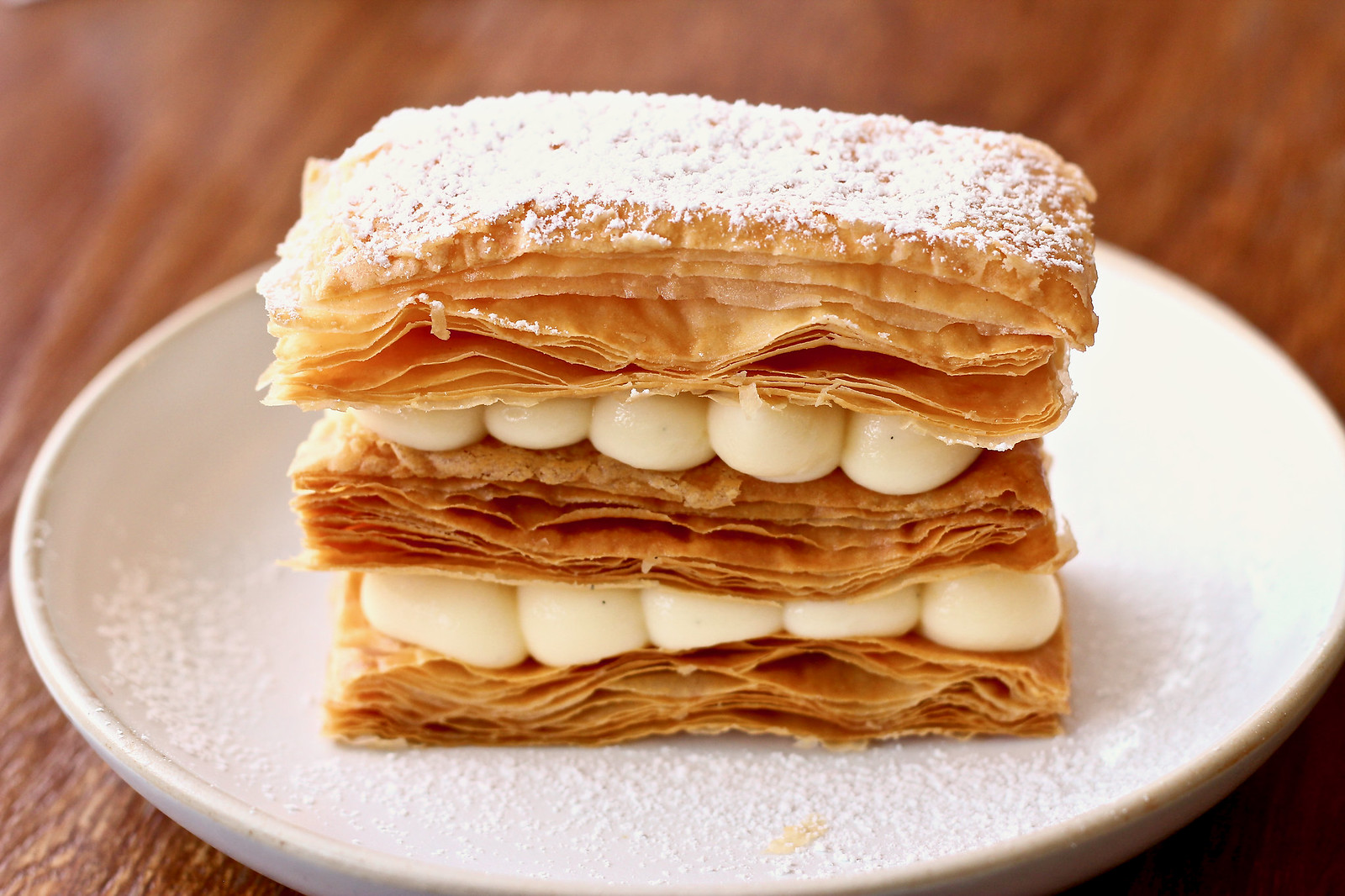The photograph captures a delicate, rectangular dessert showcased on a small white plate resting on a dark brown wooden table. The dessert is constructed from three layers of light brown, flaky puff pastry, each generously dusted with powdered sugar. Between the layers, rows of marshmallows or vanilla cream, piped to be as wide as a thumb, form two layers, totaling five lines per layer. The bottom layer begins with multiple sheets of this puff pastry, while the topmost layer is thicker and more robust. The powdered sugar not only decorates the top but also lightly scatters onto the plate, adding to the elegant presentation. The background is softly blurred, emphasizing the intricate and refined nature of this meticulously crafted dessert.